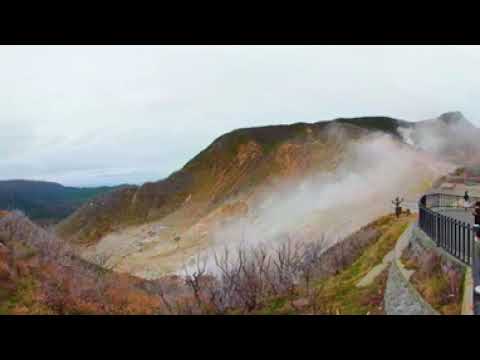The image depicts a vintage or slightly faded photograph capturing a mountainous landscape. The central focus is a colorful mountain, adorned with vivid greens, oranges, and purples, indicating a rich array of vegetation. Splashes of white hint at mist, clouds, or possibly snow, reflecting the high altitude or the presence of natural phenomena like fog or wildfire smoke. The sky above is hazy and overcast, contributing to the image's muted and aged appearance.

In the bottom right corner, a circular fence or guardrail, likely black, encloses a public viewing area or parking lot, where people are seen standing and observing the scenery. This fence serves as a safety barrier, preventing access to the steep drops of the mountainous terrain. The mountain itself features a flat plateau descending to the left, with additional mountain ranges visible in the distance, shaded in purple hues.

Low-hanging clouds drift among the mountains, adding to the ethereal atmosphere. The natural colors span a broad palette, from greenery to shades of orange and purple, as well as white, black, and hints of yellow and red. The scene captures an outdoor vista during the day, possibly in fall or winter, offering a panoramic view of the diverse and scenic mountain range.